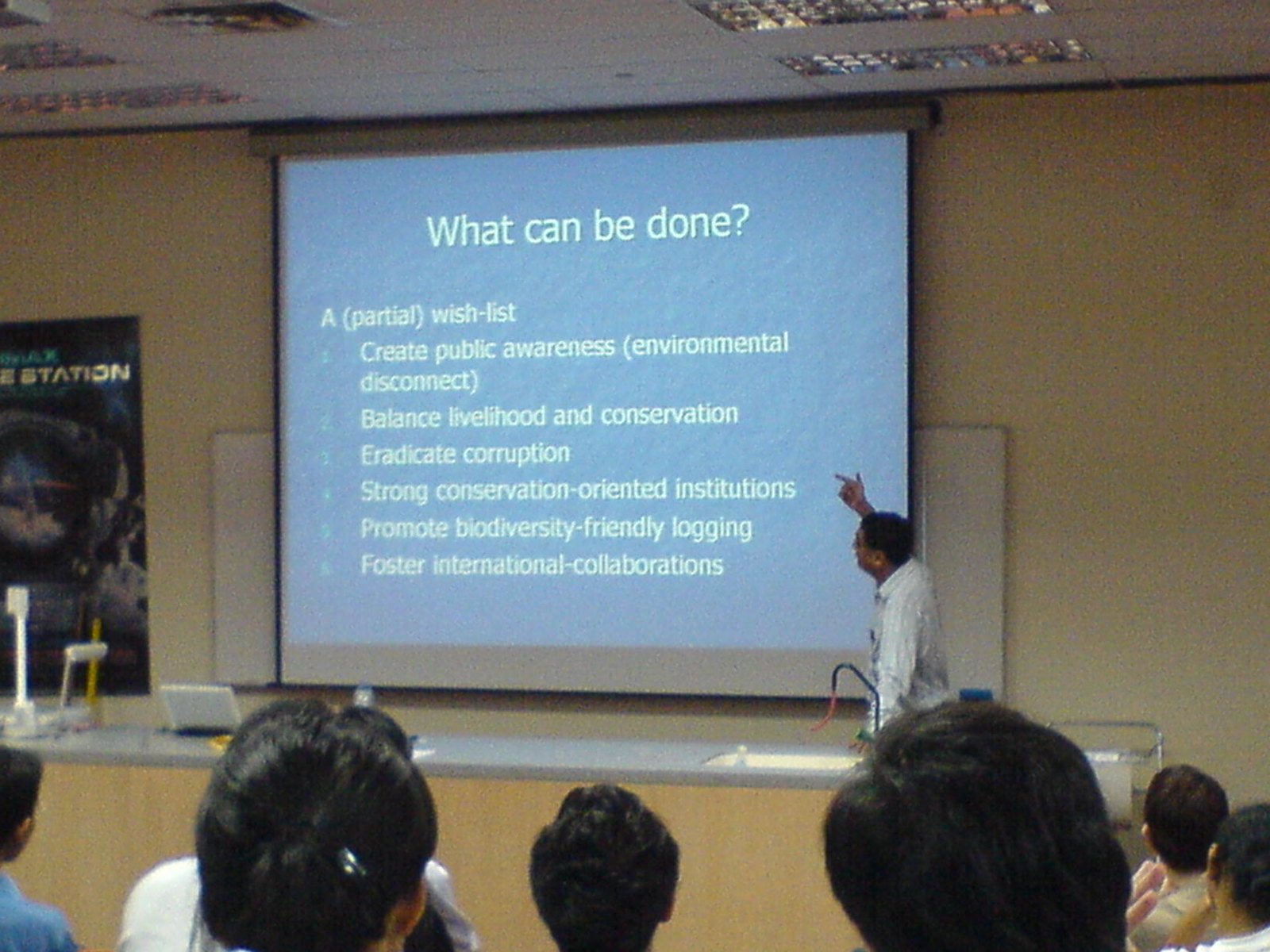In this classroom photograph taken from a student's perspective, a teacher stands beside a pull-down projector screen, attentively pointing to words on the slideshow. The man is dressed in a white button-down shirt and is intently focusing on his presentation. The projected screen displays a blue background with white text, headered by the question, "What can be done?" followed by the subtitle "A partial wish list." The list includes bullet points such as creating public awareness, balancing livelihood and conservation, eradicating corruption, fostering strong conservation-oriented institutions, promoting biodiversity-friendly logging, and encouraging international collaborations. In the foreground, the backs of students' heads can be seen, indicating their attention is fully directed towards the presentation. Additionally, a long wooden table with a grey countertop and a sink on the right-hand side is visible at the front of the classroom.